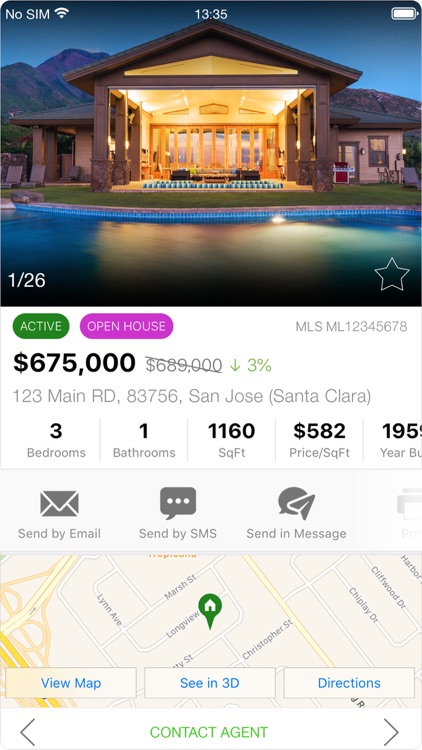In this image, set against a stark white background, the top left corner displays various pieces of technical information: "No SIM," a Wi-Fi signal icon, "13:35" (indicating the time), and a fully charged battery icon. Dominating the center of the image is a vibrant, full-color photograph of an opulent home. 

The property features an inviting swimming pool in the foreground, framed by an expansive outdoor seating area flanked by stately columns on both the right and left sides. In the distance, a majestic mountain range serves as a scenic backdrop. 

This listing is dated "1/26," and visibly includes two interactive buttons labeled "Active" and "Open House." Pertinent details follow, including the MLS number "ML12345678," the current asking price of $675,000 in bold black text, alongside a previous price of $689,000 shown crossed out with a red downward arrow indicating a 3% reduction. 

The address is cited as "123 Main Road, San Jose, Santa Clara, 83756." The home boasts three bedrooms and one bathroom, offering a total of 1160 square feet of living space, equating to a price of $582 per square foot.